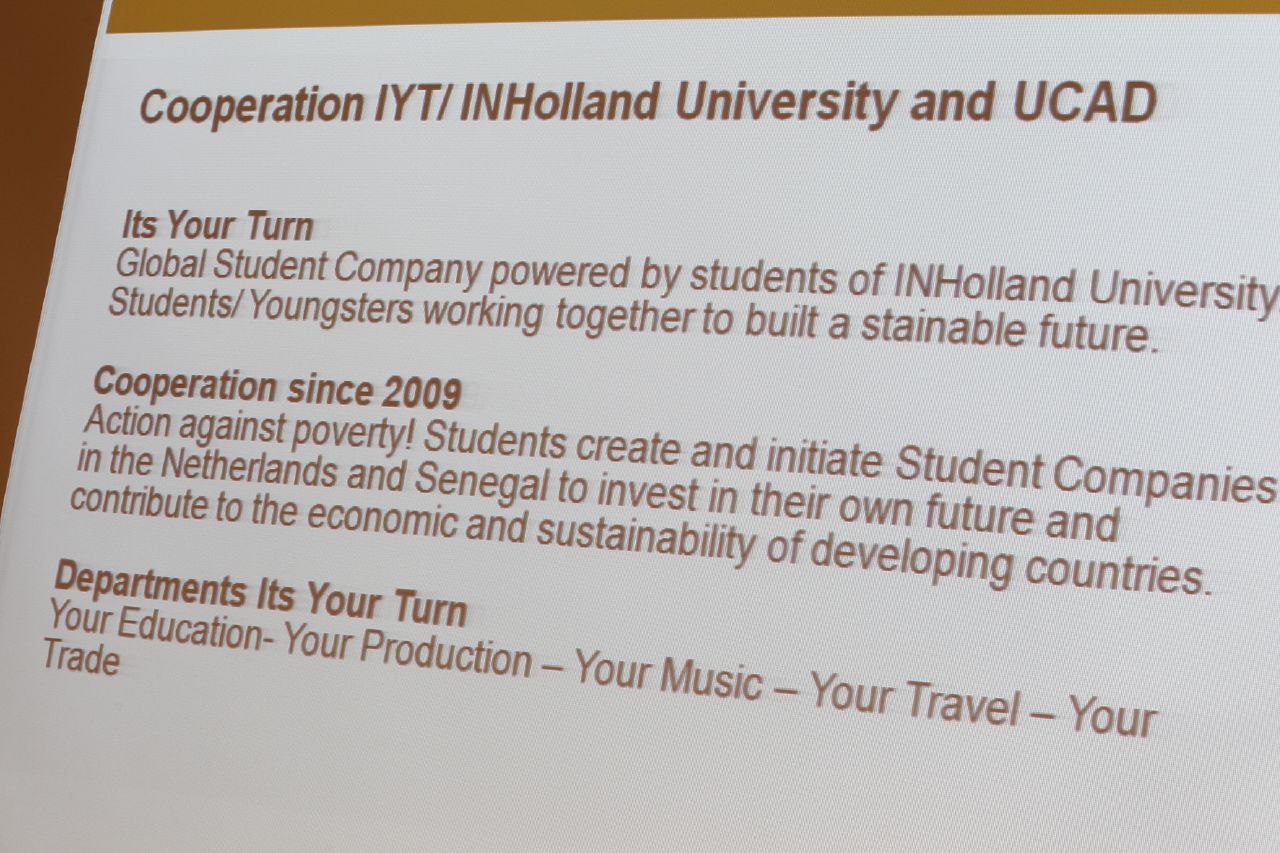The image features a page with a light gray, lavender-ish background and black text. At the top, in bold print, it says, "Cooperation IYT / IN Holland University and UCAD." Below that, the text "It's Your Turn" appears in smaller bold print. The subsequent line reads in thinner font, "Global Student Company powered by students of IN Holland University," followed by, "Students / youngsters working together to build a sustainable future." Another section, starting in capital bold letters, states, "Cooperative since 2009," and below that in smaller print, "Action against poverty!" The content explains that "Students create and initiate student companies in the Netherlands and Senegal to invest in their own future and contribute to the economy and sustainability of developing countries." Further down, in bold capital letters, it reads, "Departments. It's Your Turn," with subpoints listing: "Your education — your production — your music — your travel — your trade." The page appears to be a photograph taken at an angle, possibly from a digital screen.